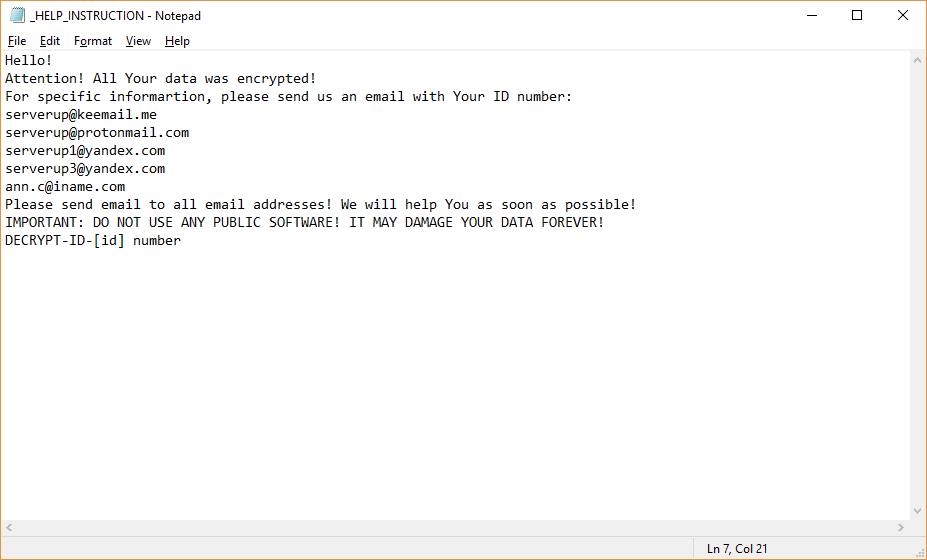The image depicts a screenshot of the Notepad application on a Windows operating system. At the top of the application, the traditional menu bar is visible, featuring options like File, Edit, Format, View, and Help. Above this menu bar, there is an icon of a blue notepad, with the text "HELP_INSTRUCTION - NOTEPAD" displayed in capital letters beside it. Towards the top-right corner of the application, the standard window control buttons for minimizing, maximizing, and closing the window are visible. 

The screenshot is highlighted by an orange rectangle around the Notepad window. Within the text area of the Notepad application, a message is displayed in plain text form. The content of the message is as follows:

```
HELLO!
ATTENTION!
ALL YOUR DATA WAS ENCRYPTED!
For specific information, please send us an email with your ID number.

server_up@keemail.me
server_up@protonmail.com
server_up1@yandex.com
server_up3@yandex.com
.c@iname.com

Please send email to all email addresses. We will help you as soon as possible!
IMPORTANT: DO NOT USE ANY PUBLIC SOFTWARE!
IT MAY DAMAGE YOUR DATA FOREVER!
Decrypt-ID-open brackets, your ID, close brackets and number.
```

Additionally, at the bottom right-hand corner of the image, the cursor's position is marked as "Ln 7, Col 21," indicating that the cursor is located on line 7, column 21 of the text document.